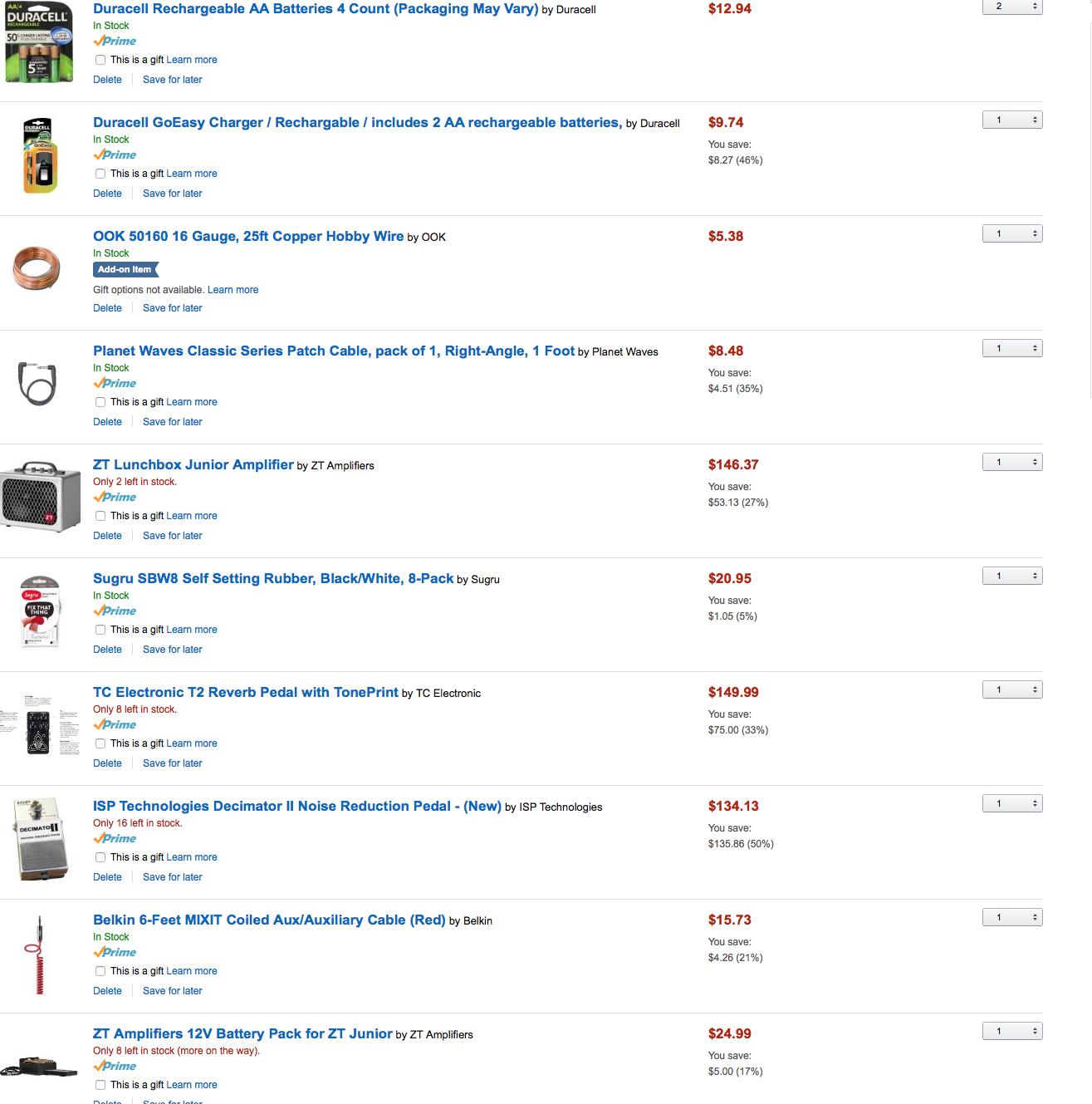The image showcases a detailed screenshot of an Amazon cart filled with various products and their respective details. Each product entry comprises the item’s image, name, seller, price, savings, stock status, and quantity selectors. Here’s a breakdown of the highlighted items in the cart:

1. **Duracell Rechargeable AA Batteries, 4-Count**:
   - **Image Description**: Photo of a 4-pack package of Duracell batteries.
   - **Text Details**: The product name in blue, with "Duracell" in black, priced at $12.94 in red. An orange checkmark indicates that it is available with Amazon Prime. Quantity set to 2 with up and down arrows for adjustment.
   
2. **Duracell EasyGo Charger with 2 AA Rechargeable Batteries**:
   - **Image Description**: Photo of the charger.
   - **Text Details**: Product name in blue with "Duracell" in black text. Priced at $9.74, showing a savings of $8.27 (46%). Quantity set to 1.
   
3. **OOK 50160 16 Gauge, 25 FT Copper Hobby Wire**:
   - **Image Description**: Photo of the copper wire.
   - **Text Details**: Product name in blue with "OOK" in black. Priced at $5.38 with a quantity of 1.
   
4. **Planet Waves Classic Series Patch Cable, Right Angle, 1 Foot**:
   - **Image Description**: Photo of the patch cable.
   - **Text Details**: Product name in blue with "Planet Waves" in black. Priced at $8.48, showing a savings of $5.41. Quantity set to 1.
   
5. **ZT Lunchbox Junior Amplifier**:
   - **Image Description**: Photo of the amplifier.
   - **Text Details**: Product name in blue with "ZT Amplifiers" in black. Priced at $146.37, showing a savings of $53.13 (27%). Quantity set to 1. Only two left in stock.
   
6. **Sugru SBW8 Self-Setting Rubber, Black/White, 8-Pack**:
   - **Image Description**: Photo of the Sugru pack.
   - **Text Details**: Product name in blue with "Sugru" in black. Priced at $20.95. Quantity set to 1.
   
7. **TC Electronic Reverb Pedal**:
   - **Image Description**: Photo of the reverb pedal.
   - **Text Details**: Product name in blue with "TC Electronic" in black. Priced at $149.99, showing a savings of $75. Eight left in stock. Quantity set to 1.
   
8. **ISP Technologies Decimator II Noise Reduction Pedal**:
   - **Image Description**: Photo of the noise reduction pedal.
   - **Text Details**: Product name in blue with "ISP Technologies" in black. Priced at $134.13, showing a savings of $135 (50%). Quantity set to 1. Sixteen left in stock.
   
9. **Belkin MIXIT Coiled AUX/Auxiliary Cable, 6 Feet**:
   - **Image Description**: Photo of the cable.
   - **Text Details**: Product name in blue with "Belkin" in black. Priced at $15.73, showing a savings of $4.26 (21%). Quantity set to 1.
   
10. **ZT Amplifiers 12V Battery Pack for ZT Lunchbox Junior**:
    - **Image Description**: Photo of the battery pack.
    - **Text Details**: Product name in blue with "ZT Amplifiers" in black. Priced at $24.99, showing a savings of $5 (17%). Quantity set to 1. Eight left in stock.

Each product entry includes interactive elements such as "Save for Later" and "This is a gift" options, with instructive icons and checkmarks indicating Amazon Prime eligibility.